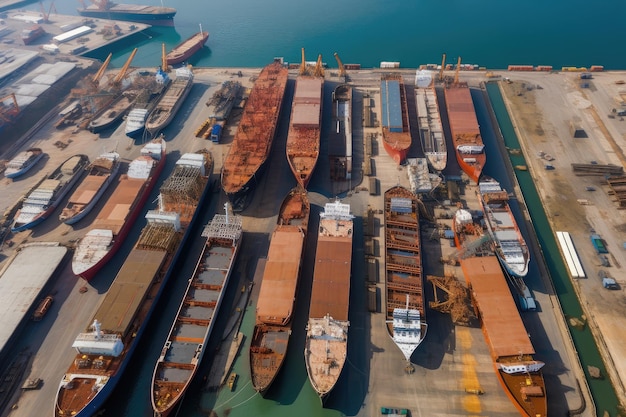The image showcases an expansive shipyard from an aerial perspective, featuring approximately 20 to 25 various shipping vessels, ranging from large to small, including barges and cargo ships, many of which appear old and rusted. The vessels are situated in dry dock, attached to a segmented cement platform interspersed with narrow strips of water. The background reveals a serene body of vibrant blue water, possibly an ocean, bay, or one of the Great Lakes. Although most ships are dry-docked and seemingly undergoing repairs or awaiting disposal, a couple of vessels are visible in the water, signifying they may still be actively used. The ships, characterized by long structures designed to accommodate crates and containers, portray a scene of industrial stillness against the contrasting hues of blue and hunter green waters.